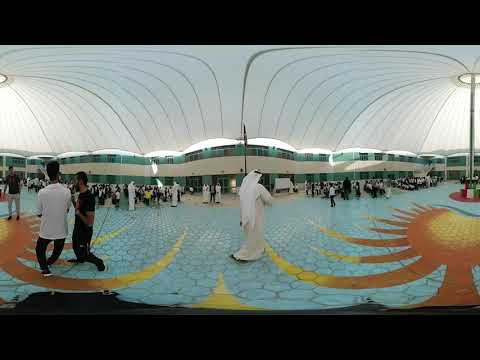In this detailed image, we observe a bustling indoor setting, possibly in Saudi Arabia, evoking an atmosphere of a significant cultural or social gathering. The scene is dominated by a vast white canvas roof with structure beams, extending across the entire space and allowing ample light to permeate. The floor is adorned with intricate hexagonal tiles in a vibrant palette of light blue, red, and yellow, depicting a sun design with golden rays.

Central to the image is a man dressed in traditional white Arab robes and a headdress secured with a black band, walking with his back to the camera under the expansive white canopy. This main figure is surrounded by numerous other individuals dispersed throughout the area; some are walking, while others are sitting or conversing.

To the left, two men stand out due to their contrasting attire: one in a white sport coat, black pants, and sneakers, the other in all black. A glass-enclosed terminal or building with green-tinted glass walls and a continuous white section across its expanse can be seen in the background, further framing the lively and colorful scene of this substantial event.